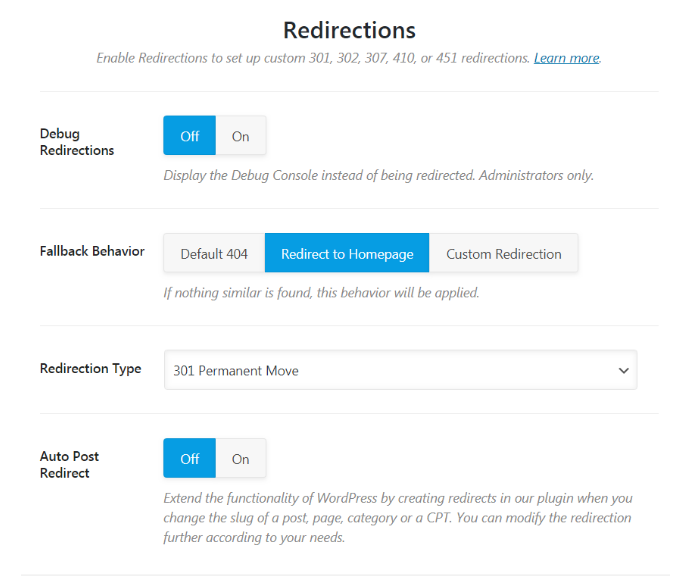The image displays a section of a WordPress website editor interface focused on managing redirections. At the top, there's a heading titled "Redirections," accompanied by a prompt encouraging users to enable redirections for custom 301, 302, 307, 410, or 451 redirects. A blue text link labeled "Learn More" is available for additional information.

Below this, there are several configurable options:

1. **Debug Redirections**:
   - Toggle buttons labeled "Off" or "On," with the "Off" option currently selected. 
   - A comment beside this feature clarifies its purpose: "Display the debug console instead of being redirected (administrators only)."

2. **Fallback Behavior**:
   - Three radio buttons labeled "Default 404," "Redirect to home page," and "Custom redirection."
   - The "Redirect to home page" option is selected, indicated by its blue-highlighted state.

3. **Redirection Type**:
   - A dropdown menu is present, showing "301 Permanent Move" as the selected option. The other options in the dropdown are not visible in the image.

4. **Auto Post Redirect**:
   - Toggle buttons labeled "Off" or "On," with "On" being the selected state.
   - An accompanying description reads: "Extend the functionality of WordPress by creating redirects in our plugin when you change the slug of a post, page, category, or CPT. You can modify redirection further according to your needs."

The interface clearly facilitates the setup and customization of various redirection rules within a WordPress environment.